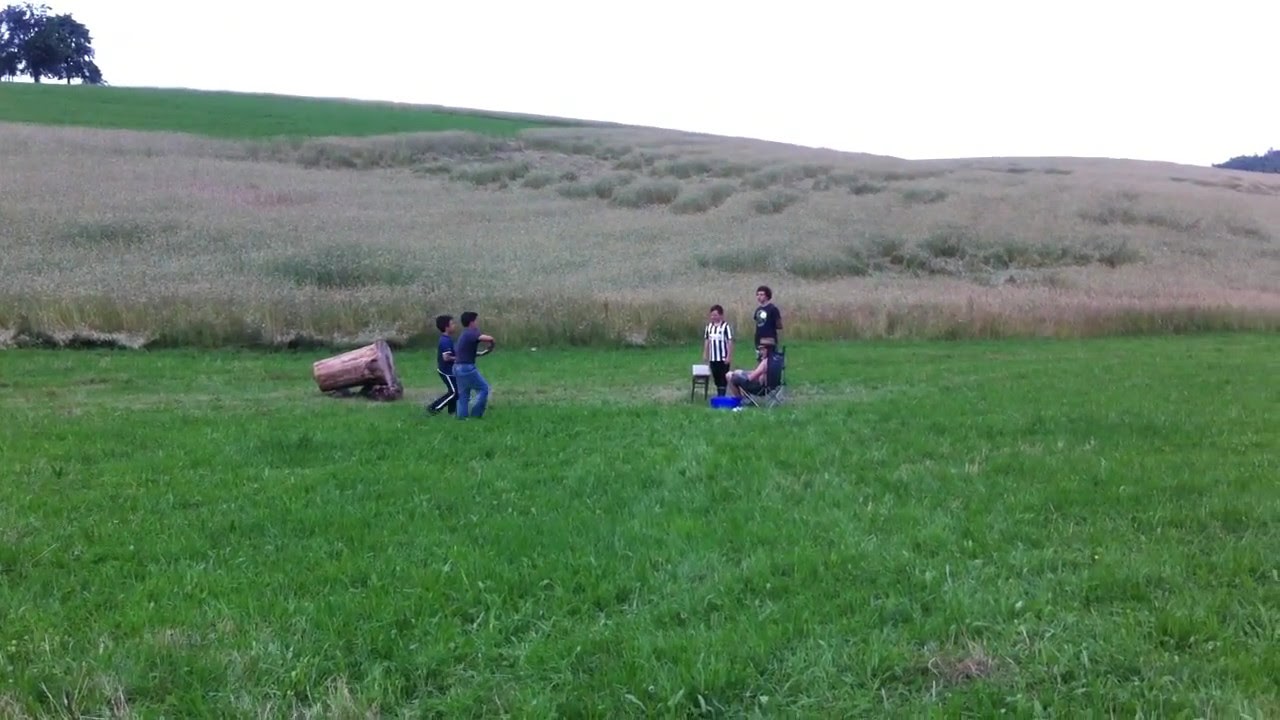The photo captures an outdoor scene in a large grassy field that has been mowed, with patches of tall brown grass or wheat in the background. Five people, including three kids and two adults, are in the center of the image. Two of the kids, who are wearing blue jeans and blue t-shirts, stand close together with a tree stump nearby. The third child, in a black t-shirt, stands across from them. One adult, dressed in a black and white referee-style shirt and black pants, stands next to the kids, possibly beside a small table or additional chair. Another adult sits in a folding camping chair. In the background, a single dark tree stands on a grassy hill under a dull, white sky. The photo is brightly lit by natural daylight, offering clear and high-quality details.